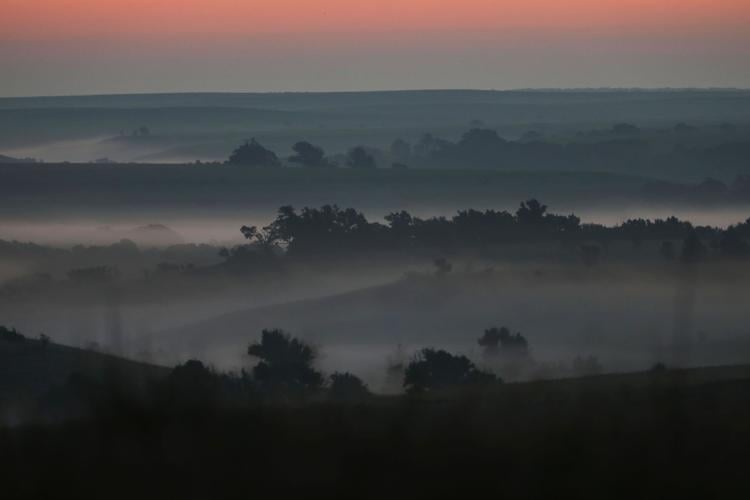The image captures an early morning landscape shrouded in mist. The sky transitions from a soft orange at the top to a dull, dusty gray below, giving way to heavy clouds that dominate the scene. The horizon features multiple rows of trees, which appear almost silhouetted against the gray mist enveloping the landscape. Though the exact terrain is ambiguous, it could be a mix of water bodies or mountain ranges with peaks and valleys, adding to the misty, ethereal quality of the view. Lower in the picture, the mist thickens, almost blending into the nearly black foreground, creating a stark contrast. The overall ambiance is hazy, with floating clouds of smoke-like mist that imbue the image with a sense of tranquil melancholy, captured as the day shifts towards night or dawn.